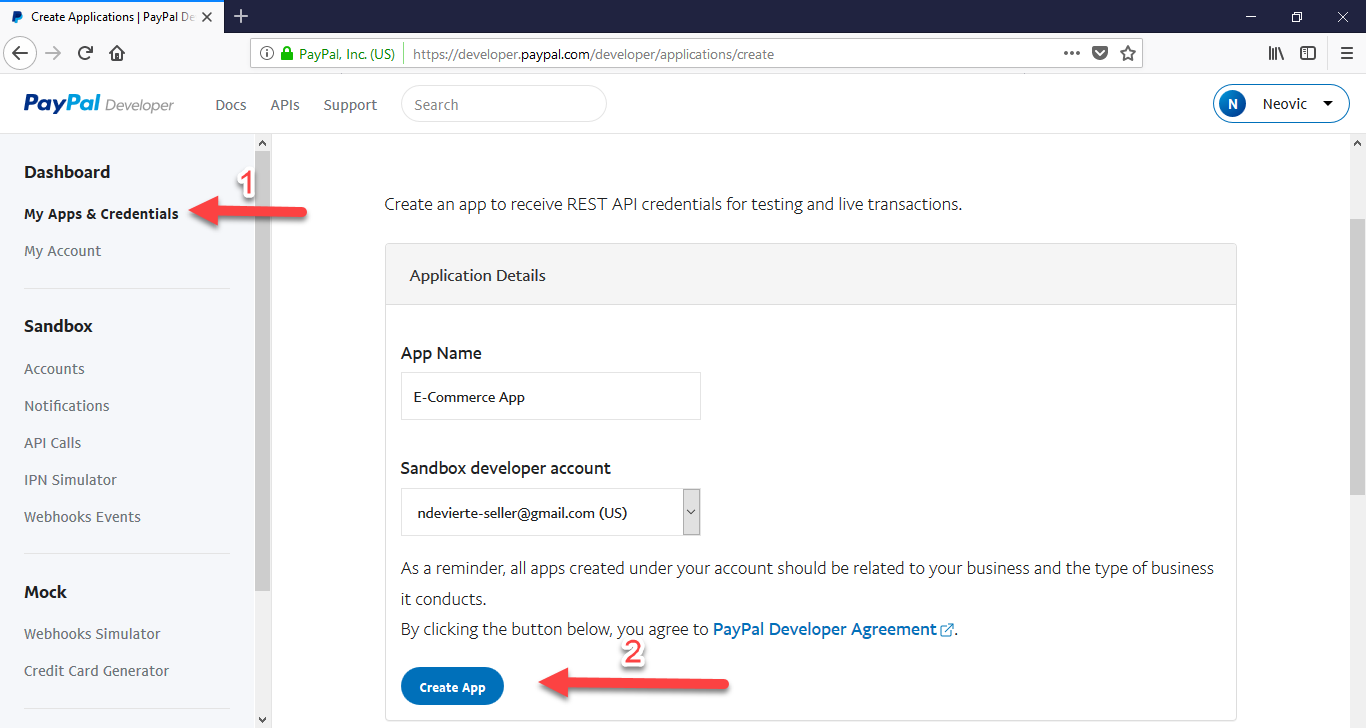**Caption:**

The image displays the "developer.paypal.com/developer/applications/create" webpage. The URL is prominently shown at the top, followed by the label "PayPal Inc USA" in green alongside a secure lock icon indicating a secure connection. The page header reads "Create Application," and there are tabs for "PayPal Developer," "Docs," "APIs," and "Support." Below these tabs is a search bar.

On the right side of the page, a blue button with a pull-down menu is visible, labeled "Nevoc" (N-E-O-V-I-C), and a blue circle with an "N" icon beside it. The left side features a navigation menu, which includes:
- Dashboard
- My Apps & Credentials (highlighted with a red arrow and a number "1")
- My Account
- Sandbox
- Account Notifications
- API Calls
- IP Simulator
- Webhooks
- Events
- Mock Webhooks
- Simulator
- Credit Card Generator

Below the menu is a section that reads: "Create an app to receive REST API credentials for testing and live transactions." The application details displayed include:
- App Name: "e-commerce app"
- Sandbox Developer Account: "ndeviert-seller@gmail.com" (US)

A reminder at the bottom of the page advises that all apps created under the account should be related to the user's business and the nature of their operations.